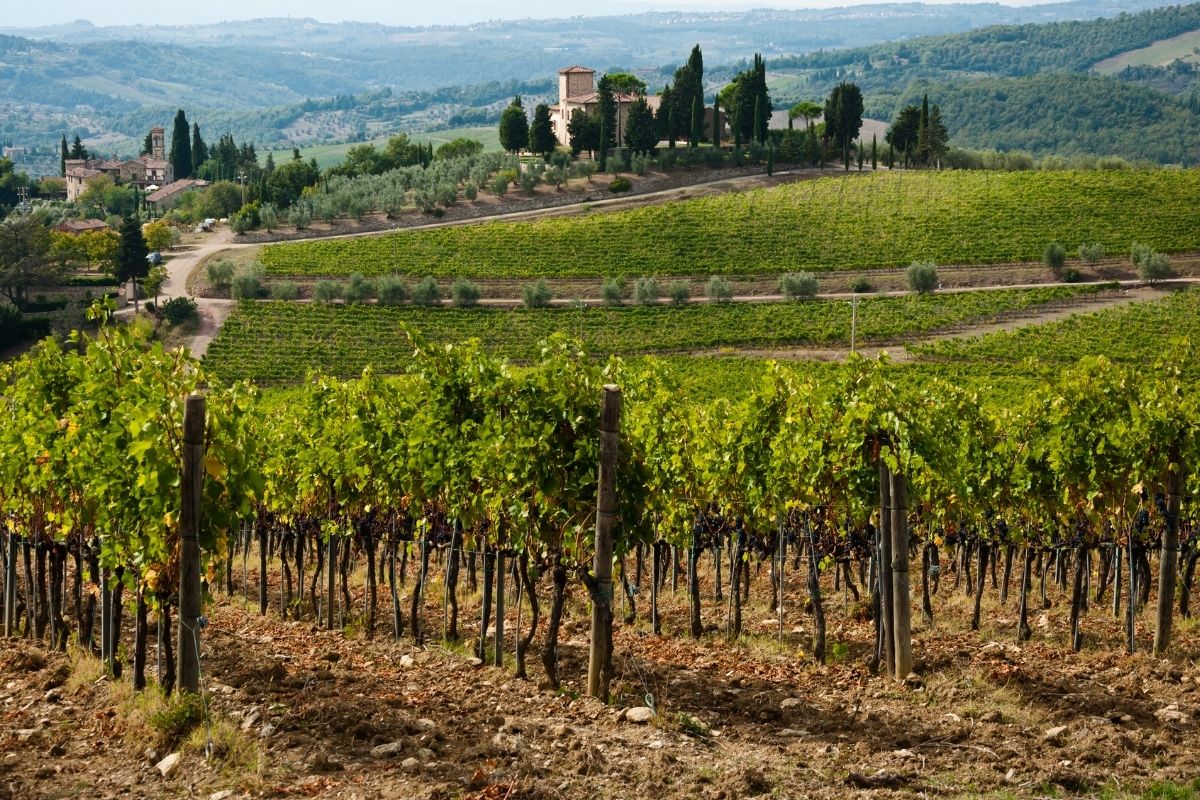This realistic photo captures an idyllic vineyard landscape, reminiscent of the Italian countryside. In the foreground, there are meticulously arranged rows of grapevines, each row punctuated by sturdy posts and abundant with lush, green foliage at the top. The vineyard stretches across a dirt field, creating a textured patchwork of greenery and earth.

In the distance, the landscape unfolds into rolling, grass-covered hills, adorned with patches of open space that contrast with the vibrant green. Amidst these hills are two notable buildings: one, on the left, resembles a mini castle or elaborate home surrounded by trees, and the other, slightly farther down in the valley, features a mini tower and is also bordered by trees. This second building is centrally located within the image. Both structures evoke the charm of wineries, enhancing the vineyard's romantic and rustic appeal.

Roads meander up to these homes, weaving through the verdant hills and connecting the various elements of this serene rural tableau. Overall, the image vividly captures the essence of a vineyard nestled in a picturesque, rolling landscape.